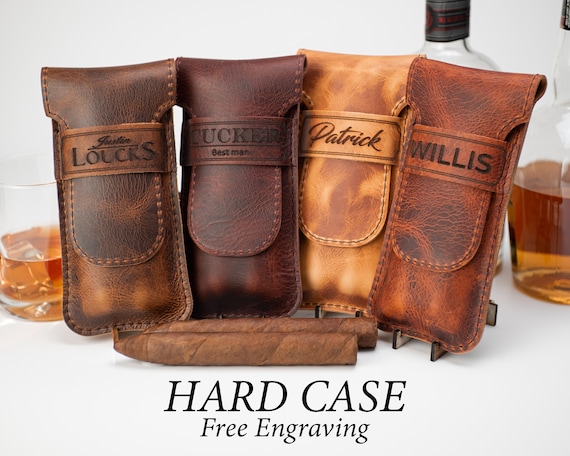This is a detailed photo advertisement showcasing four leather cigar cases, each personalized with engravings such as "Justin Louks," "Tucker Best Man," "Patrick," and "Willis." The cases vary in shades of brown, from light tan to dark brown, and each features a flap that tucks into a strap. Positioned at the bottom center of the image, bold black lettering reads "HARD CASE" with "FREE ENGRAVING" right below it. The backdrop is a stark white, providing a clean and minimalistic contrast against the warm tones of the leather. In the foreground, two brown cigars are placed in front of the cases, adding to the luxurious appeal. A glass, half-filled with what appears to be whiskey, sits to the left side of the image, while behind that, there is a half-filled whiskey bottle. These elements together create a sophisticated and elegant ambiance, ideal for the targeted advertising of these customizable leather cigar cases.